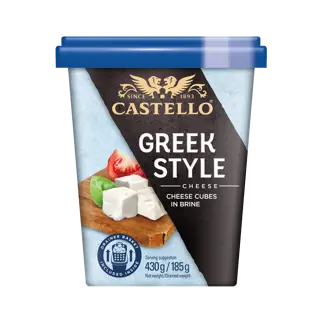This advertisement features a modern plastic container of Greek-style cheese cubes in brine from the brand Castello, spelled K-A-S-T-E-L-L-O. The container has a trapezoidal, tapered rectangular shape with straight edges. The bottom is shorter than the top, and it has a blue plastic lid with a two-tier design, featuring a square portion and a thicker lip around the edge. The main surface of the container is a baby blue color with a brown diagonal band running from the top left to the lower right, featuring the Castello logo, which includes golden lettering and an emblem of angel wings with a lion's head. The text on the brown band reads "Greek-style cheese, cheese cubes in brine" and states "since 1893." Just off to the left of the text, there is a rustic wooden cutting board illustrated with cheese cubes, tomato slices, and what looks like a piece of avocado. The nutritional information is displayed in dark blue text on a white background at the lower right corner of the container. The container size is labeled as 430 grams. All of these elements are set against a white background, emphasizing the clean and modern design of the product packaging, which would typically be found in a grocery store.